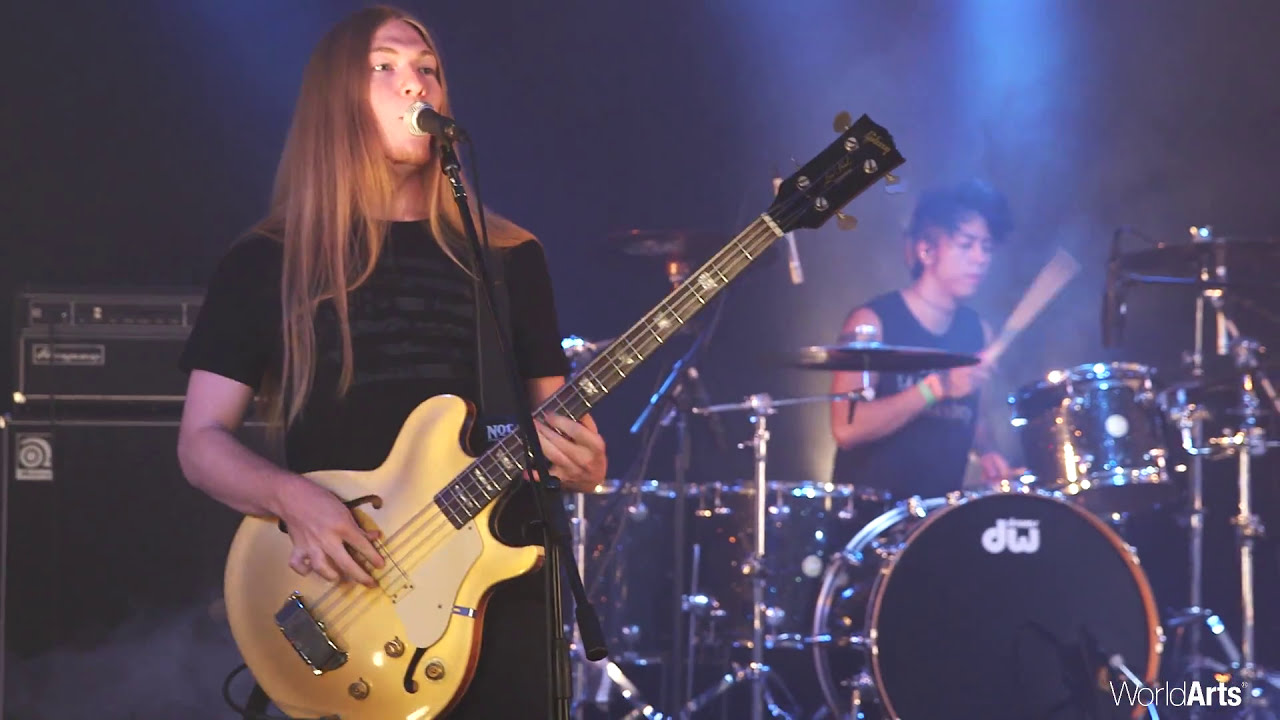The image depicts a vibrant live concert performance featuring two musicians against a smoky, dark backdrop highlighted with blue lights. On the left side of the image stands a Caucasian man with long, straight strawberry blonde hair, parted to the side and cascading to his chest. He is immersed in his performance, singing into a black microphone stand while skillfully strumming a light yellow bass guitar with a black headstock. The man is dressed in a black shirt, and his intense expression suggests his deep connection to the music.

To his right, a drummer occupies the center-right portion of the image. With short, dark hair shaved on the sides and longer on the top, he is energetically playing a large black drum set, which includes a bass drum, four toms, a hi-hat, and multiple cymbals. Dressed in a black sleeveless shirt, the drummer adds to the powerful dynamics of the performance. 

The stage setup includes an Ampeg amplifier and speaker stack to the far left, visible behind the bass player. The overall scene has a hazy, smoky atmosphere, typical of an intense rock or metal concert, with the lights creating an edgy ambiance. In the bottom right corner of the image, there is a watermark that reads "World Arts" in white font, suggesting this image might be part of promotional material or a television broadcast.